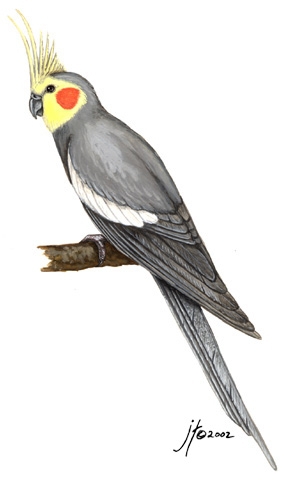This detailed painting portrays a cockatiel, a small parrot species, set against a white backdrop. The bird, shown in a left-facing side profile, exhibits predominantly gray plumage accentuated by white stripes on its wings. It possesses a yellow head adorned with a fringed crest that stands tall, and vibrant red patches on its cheeks. The cockatiel's small, downward-pointing beak and keen black eyes add to its lifelike portrayal. A long, light gray feather extends from its tail, almost reaching the painting's edge. The bird is perched on a slender, partially painted brown tree branch. The artwork is signed by the artist, J.T., and dated 2002, reminiscent of high-quality scientific illustrations akin to those found in Darwin's documentation of species.